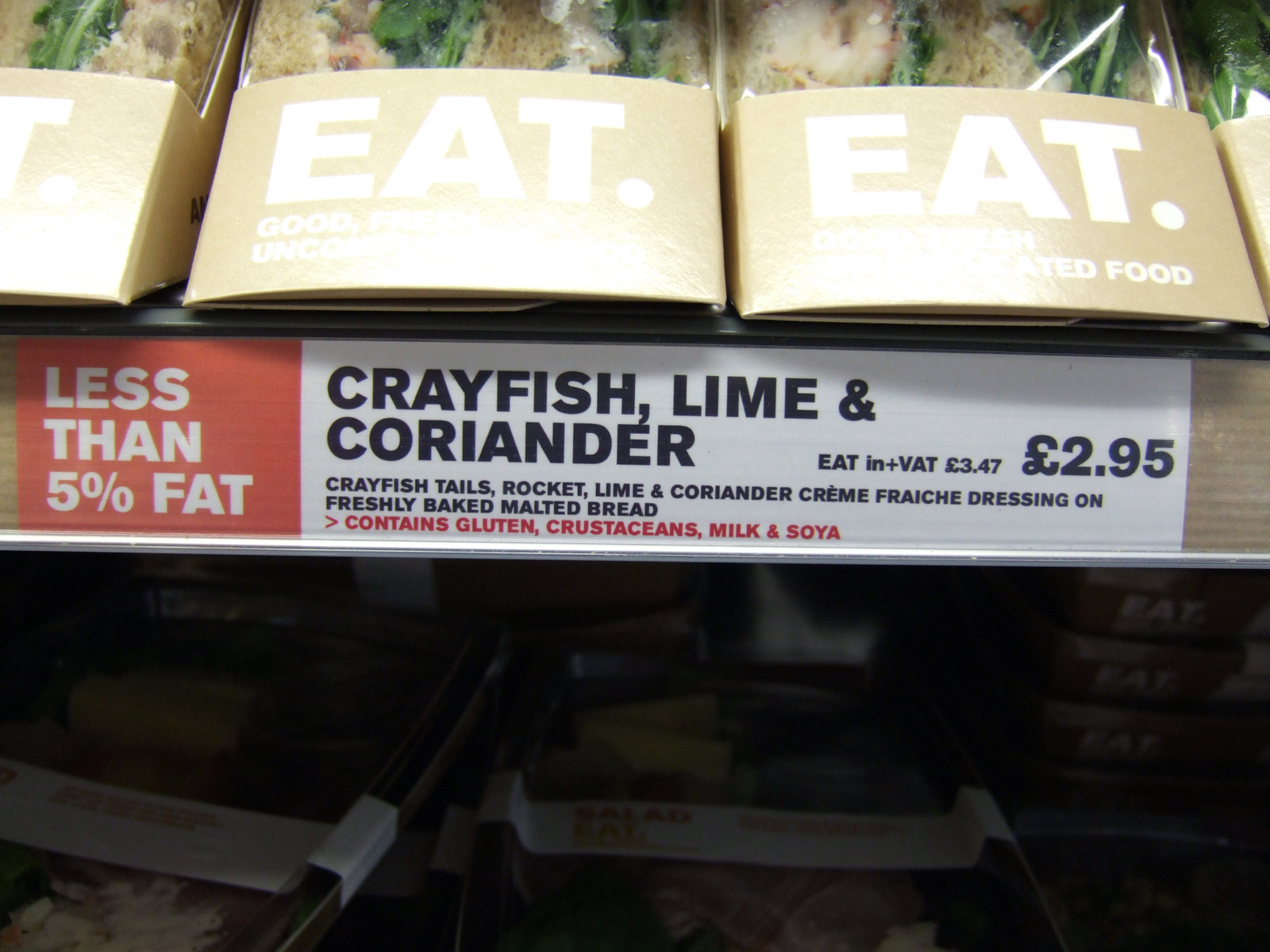The image is a color photograph in landscape orientation, depicting the interior of a European supermarket aisle focusing on a shelf of prepackaged sandwiches. The top shelf shows multiple individually wrapped sandwiches, each in boxes with a distinctive gold bottom band. Prominently displayed on each box is the word "EAT." in white lettering. Above the shelf, there is a detailed sign: on the left, an orange rectangle with white text reads "less than 5% fat." Centered on the sign, in black text against a white background, are the words "crayfish, lime, and coriander." Below this, smaller text describes the sandwich ingredients: "crayfish tails, rocket, lime and coriander cream dressing on freshly baked malted bread." To the right, the price is indicated as £2.95. The sign also warns that the sandwiches contain gluten, crustaceans, milk, and soya. The bottom half of the image is darker and shows more stacked containers, likely filled with the same type of sandwiches. Light shines down on the display, adding a focal point to the brightly lit, neatly arranged packages.